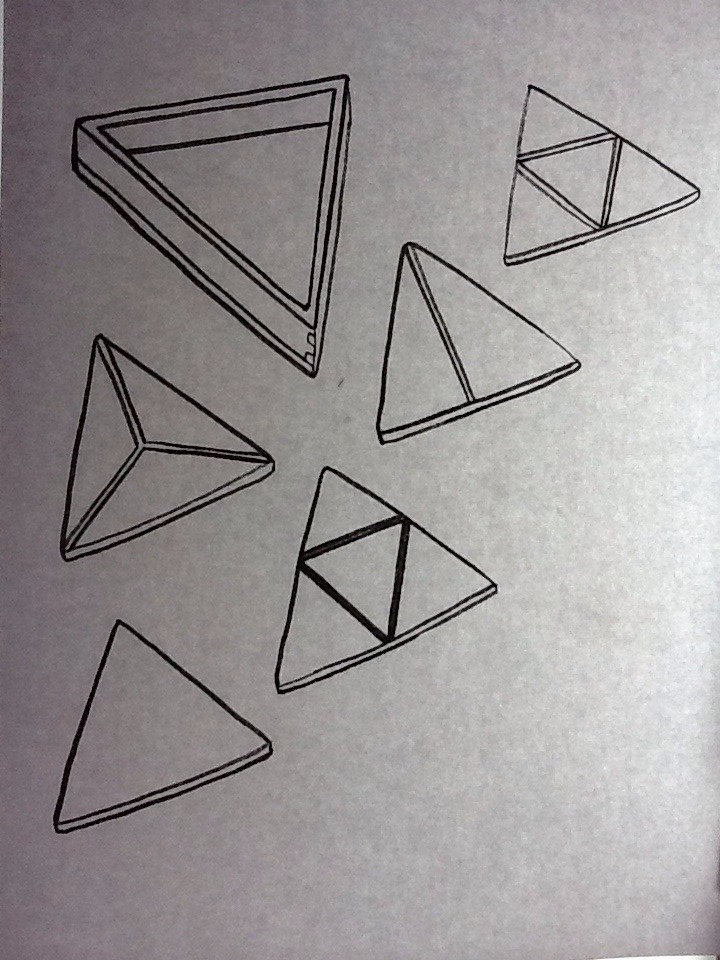This black and white drawing on a vertical white piece of paper depicts six distinct triangles, varying in style and composition. The paper appears lighter on the right side and darker towards the left, with a subtle fold in the bottom right corner that creates a small shadow. 

Starting from the top left:
1. A large triangle with a thick outline resembling a pool ball rack, open in the center.
2. A triangle split into three smaller triangles by internal lines forming an 'X' shape.
3. A plain, unadorned triangle with just a black outline.

From the bottom left:
4. A triangle with an additional triangle inside, dividing it into four smaller triangles.
5. Another triangle featuring a single vertical line from its apex to the base, creating a division.
6. Finally, a triangle containing a smaller triangle within, drawn similarly to the fourth one, dividing it into four sections.

Each triangle is distinct, showcasing different internal line configurations, with the overall arrangement creating a balanced composition on the page.